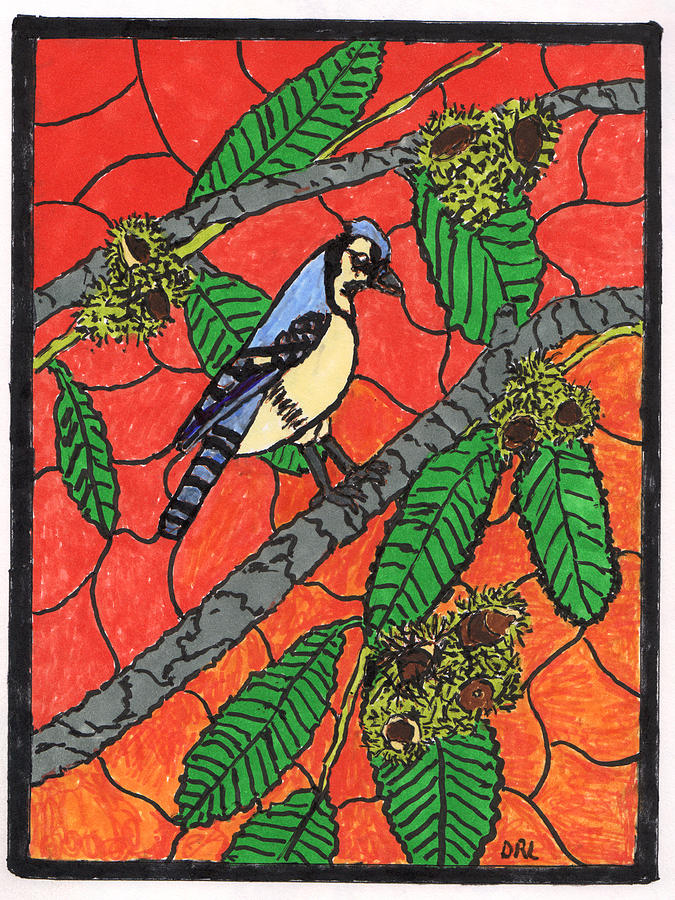This image is a detailed piece of artwork signed with the initials "DRL" at the bottom. Framed in black, the artwork appears to be made with a medium that could be watercolor or crayon. It features a vibrant blue jay with a blue crown, white face bordered by black, and blue feathers with stripes, perched centrally on a brown limb. The bird's body transitions into a white underbelly and the gray feet are gripping the branch. The branches span from right to left and are depicted in gray, surrounded by lush green leaves and clusters of what seem to be nuts or berries. The background is a striking red, segmented by linear black patterns that create a visually engaging backdrop for the natural scene. The blue jay is positioned to the side, creating a dynamic focal point against the vivid and contrasting background of red, making this artwork both captivating and detailed in its representation of nature.